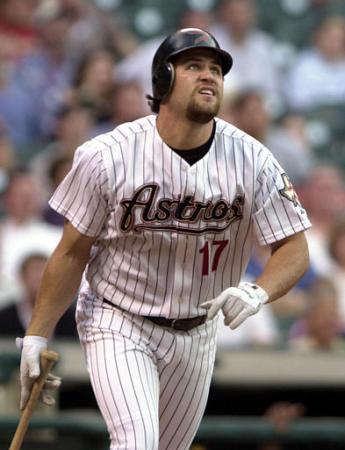The photograph captures a professional baseball player from the Houston Astros. He is wearing a white uniform adorned with vertical black pinstripes, and the word "Astros" is prominently displayed on his chest. The number 17, in red, is also visible on the front of his jersey. The player is equipped with white batting gloves on both hands and dons a black batting helmet. In his right hand, he is loosely holding a bat as he gazes skyward, likely following the trajectory of a recently hit ball. The background features a blurred image of the stadium stands filled with fans dressed in various colors, adding a dynamic atmosphere to the scene.